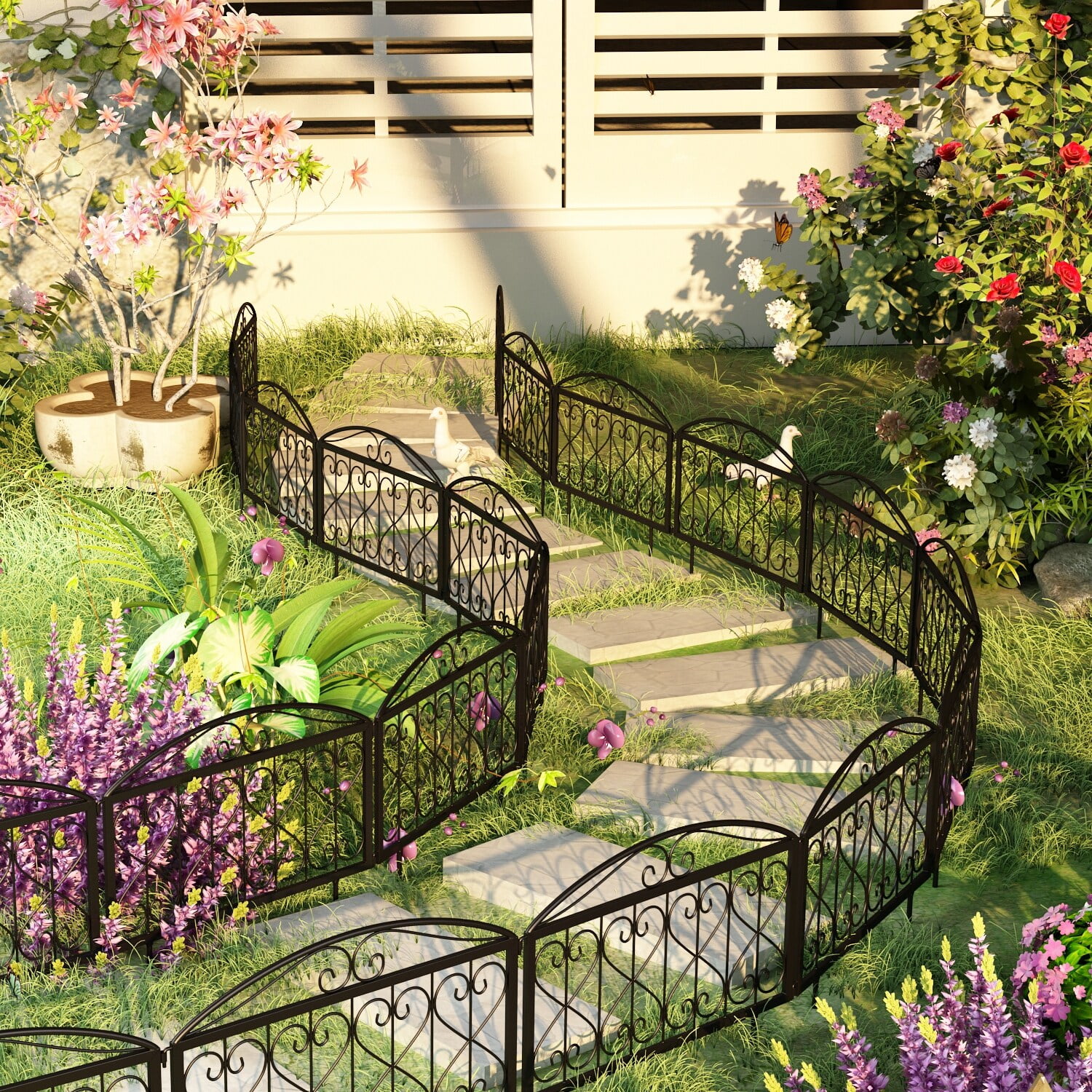The image is a detailed painting of a charming garden pathway, captured in an outdoor setting during the day. This sinuous cement path meanders in an S-shape, flowing from the background to the foreground, and flanked on either side by a black wrought iron garden fence. The path is surrounded by lush greenery, with overgrown grass and various flower bushes adding to the vibrant scene. The garden boasts a rich palette of colors, with purple irises, pink flowers, red blooms, and white blossoms scattered throughout. On the left side of the path, there is a potted plant with pink flowers sprouting from its branches. Additionally, either real or decorative ceramic doves are visible, enhancing the quaint and serene atmosphere. The path appears to lead towards a structure in the background, possibly a greenhouse or garden shed, adding an element of mystery and inviting exploration.